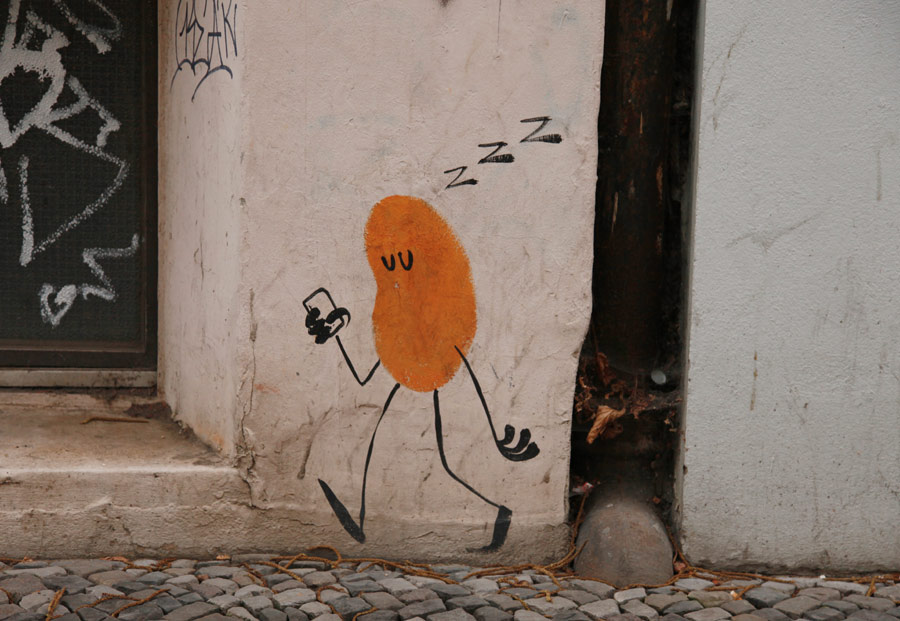The photograph provides an up-close view of a graffiti artwork outside a building, featuring a cobblestone pathway composed of granite-like rocks in shades of gray and tan that lead up to a white wall. To the left, part of a doorway is visible, just the bottom right panel, with a single step leading up to it. The wall continues with a gap before resuming on the right side, where it appears dingy with smudges and dirt marks.

Dominating the scene is a character painted on the left side of the wall, approximately one foot off the ground. The character is bean-shaped and orange, resembling a peanut or jelly bean. It has thin, spindly black lines for arms and legs, each ending in thicker black lines that represent feet and three-fingered hands. The left arm hangs down while the right arm is bent at the elbow, holding a rectangular device that suggests the character is texting.

The character has eyes depicted by two black U-shapes, giving it a sleepy appearance. This feeling is reinforced by three black Z’s above its head, symbolizing sleep. The overall impression is of a sleepwalking, cartoon-like figure. The scene is completed by a small crevice or gap between sections of the building on the right side. The environment, with its textured brick pathway and partially visible door, provides a backdrop to this whimsical graffiti figure.